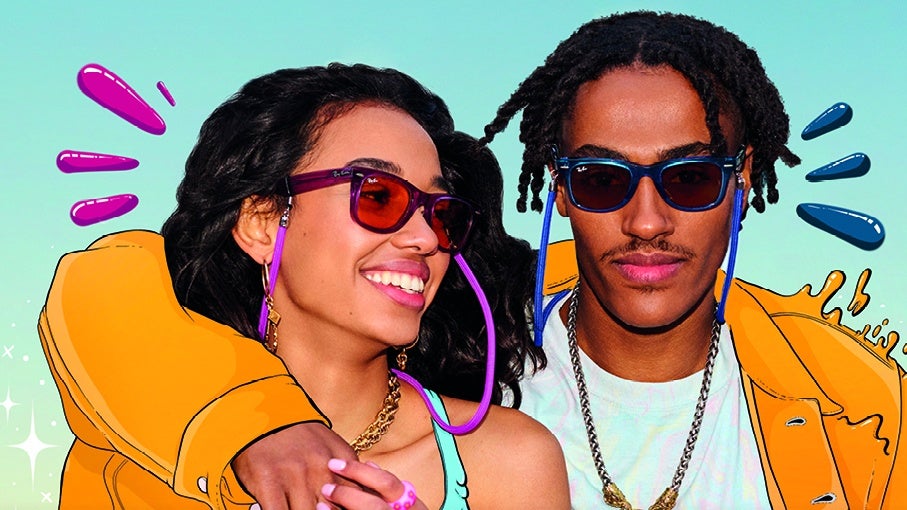A young African-American couple stands close together in a digitally painted photograph, where their real faces blend seamlessly with cartoonish, painted elements. The woman, with shoulder-length thick black hair, is leaning into the man, displaying a radiant, toothy smile as she turns her head towards him. She sports teal-blue bikini straps and a gold chain around her neck. The man, whose short dreadlocks fall just past his upper ear, is dressed in a mustard-colored, cartoonishly-painted jacket with blue and purple paint-like squirts on the shoulders. He also wears a white t-shirt, purple sunglasses, and a gold chain, with his right arm wrapped around the woman's neck and shoulder. The background features a similar digital, paint-splattered design in blue and purple hues. The man's expression is calm, with a closed-mouth smile, contrasting the woman's exuberant demeanor.